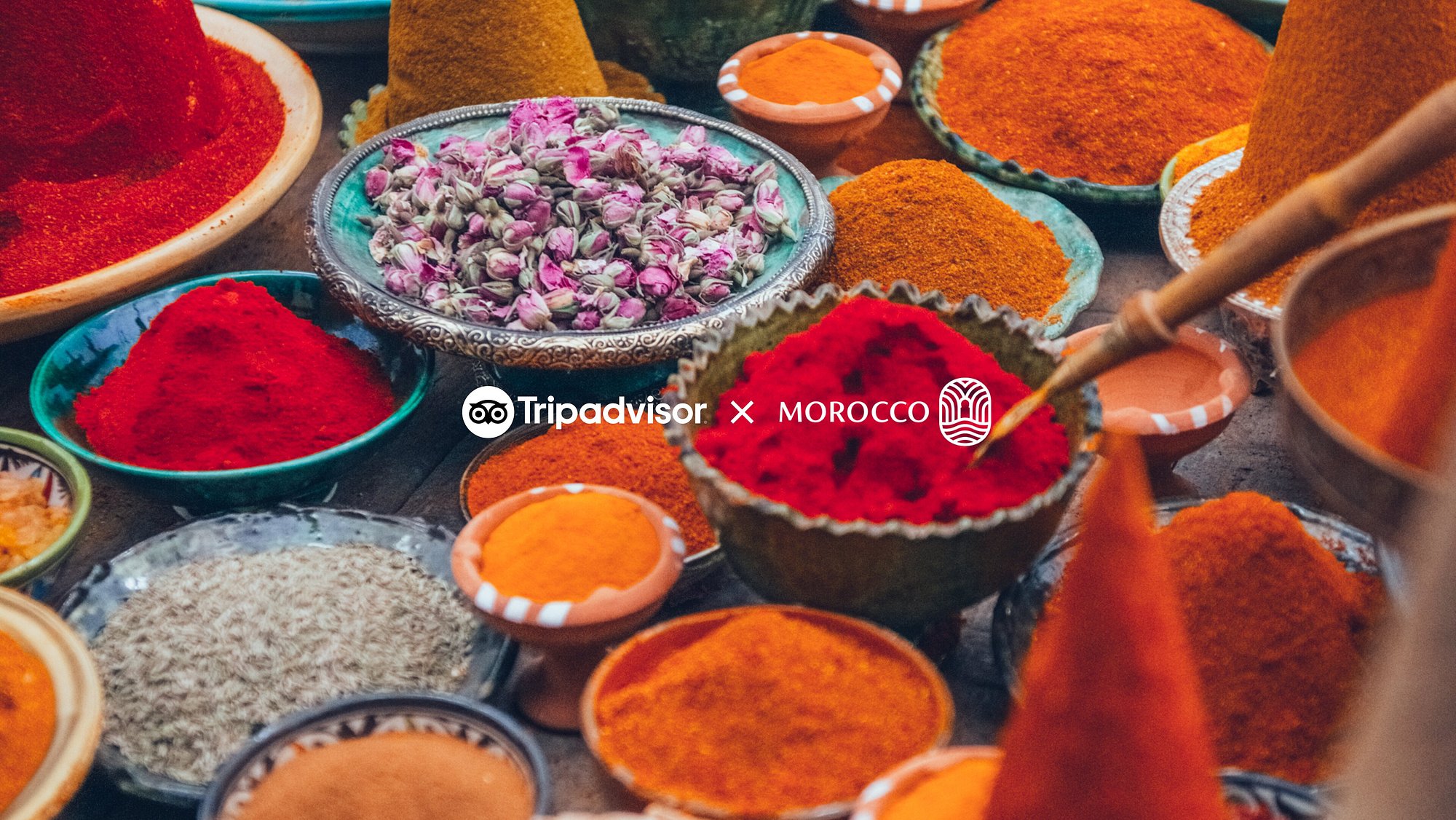This vibrant color photograph showcases an assortment of spices artfully arranged on a dark brown wooden tabletop. Central to the image is the TripAdvisor branding, featuring the distinctive owl logo to the left and the text "Times Morocco" in white, accompanied by another logo on the right. The tabletop hosts a variety of plates, some of which are intricately designed. One notable plate features an ornate silver-bordered edge with a blue center, displaying an array of purple and gray flower petals or buds. Surrounding this are bowls brimming with vivid red and orange powders, adding a burst of color to the scene. Among the collection is a terracotta bowl that stands empty, hinting at a minimalist beauty, and a black plate speckled with light brown seeds, offering a textured visual contrast. The careful composition and rich palette highlight the sensory allure of Moroccan spices.